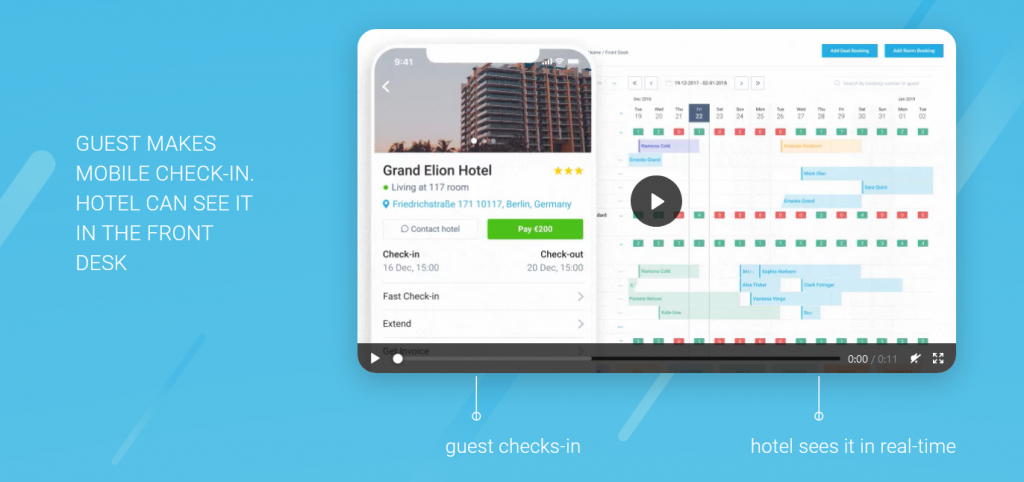This image captures a landscape-oriented screenshot from a training module on mobile hotel check-ins. In the far left section, the text indicates the process of a guest making a mobile check-in, which is visible to hotel staff at the front desk. Central to the image, inside a larger blue rectangle, is a smaller, embedded screenshot resembling a play button or video icon, suggesting a demonstration for hotel management to observe the guest's check-in via a mobile device. The embedded screenshot includes essential stay details such as check-in and check-out dates and times. There is also a mention of a calendar or schedule, though it appears too small and blurry to discern further details. The middle section features a colored image of the "Grand Elan Hotel" or "Grand Elyon Hotel," depicting a modern, high-rise building. The precise spelling of the hotel's name is unclear due to the indistinguishable third letter in the second word. Overall, this screenshot seems to serve as a visual aid to train staff on the hotel's mobile check-in system, providing both a sample view from the guest’s perspective and the hotel's side of the process.